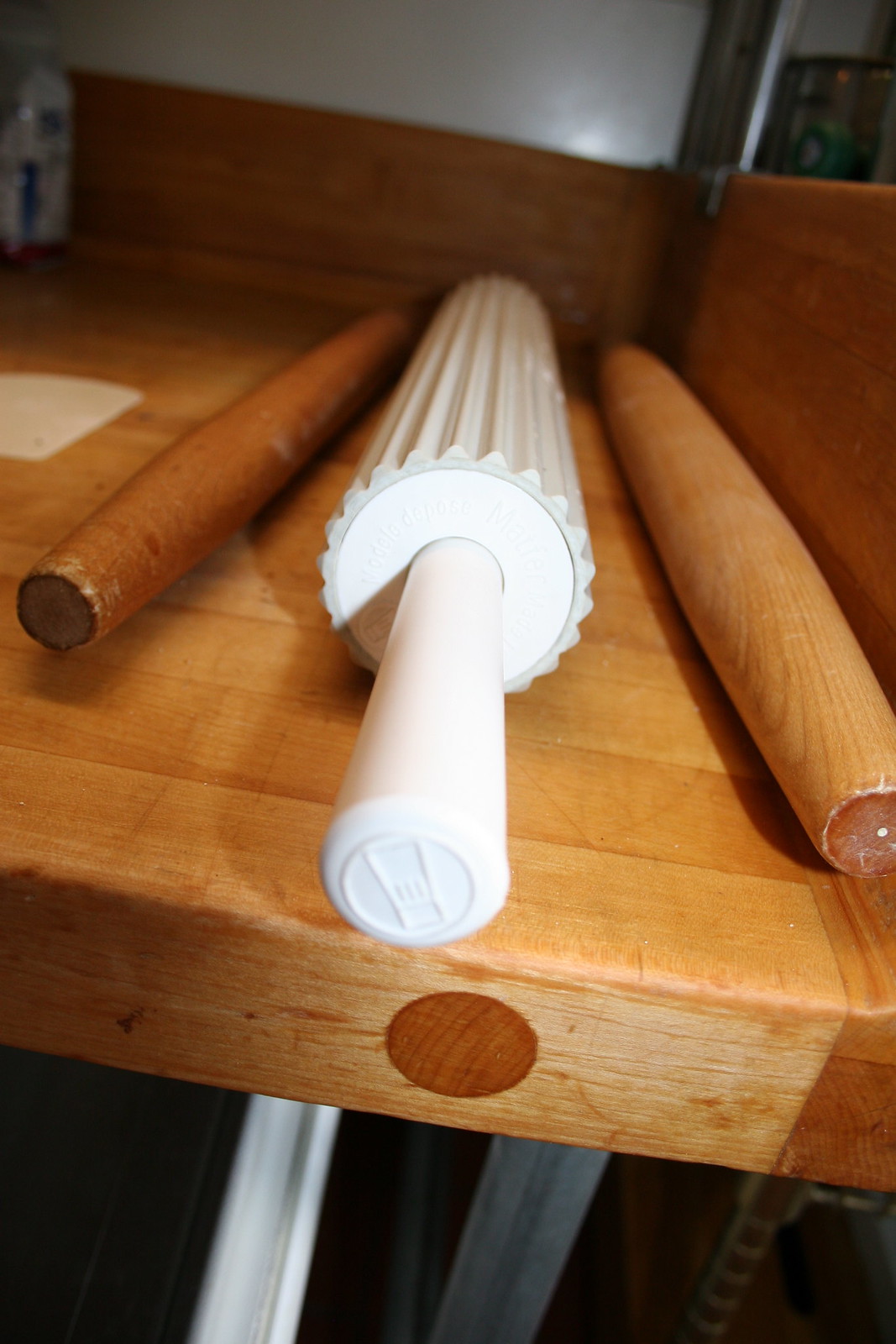This image showcases a wooden countertop, around twice as tall as it is wide, likely part of a bread-making station in a bakery. The countertop is made of light-colored wood with a narrow, approximately four-inch high wooden backboard behind it and extending to the right. On the counter are three distinctive rolling pins. The central rolling pin stands out with its white plastic construction, featuring cylindrical rivets or bumps along its surface and two side handles. Flanking this are two wooden rolling pins, both handle-less, with the one on the left being a slightly darker brown, while the one on the right is a lighter tan or beige. Additionally, in the top corners of the image, partially visible shelves hold some packaged goods, possibly including a bag of yeast on the top left.